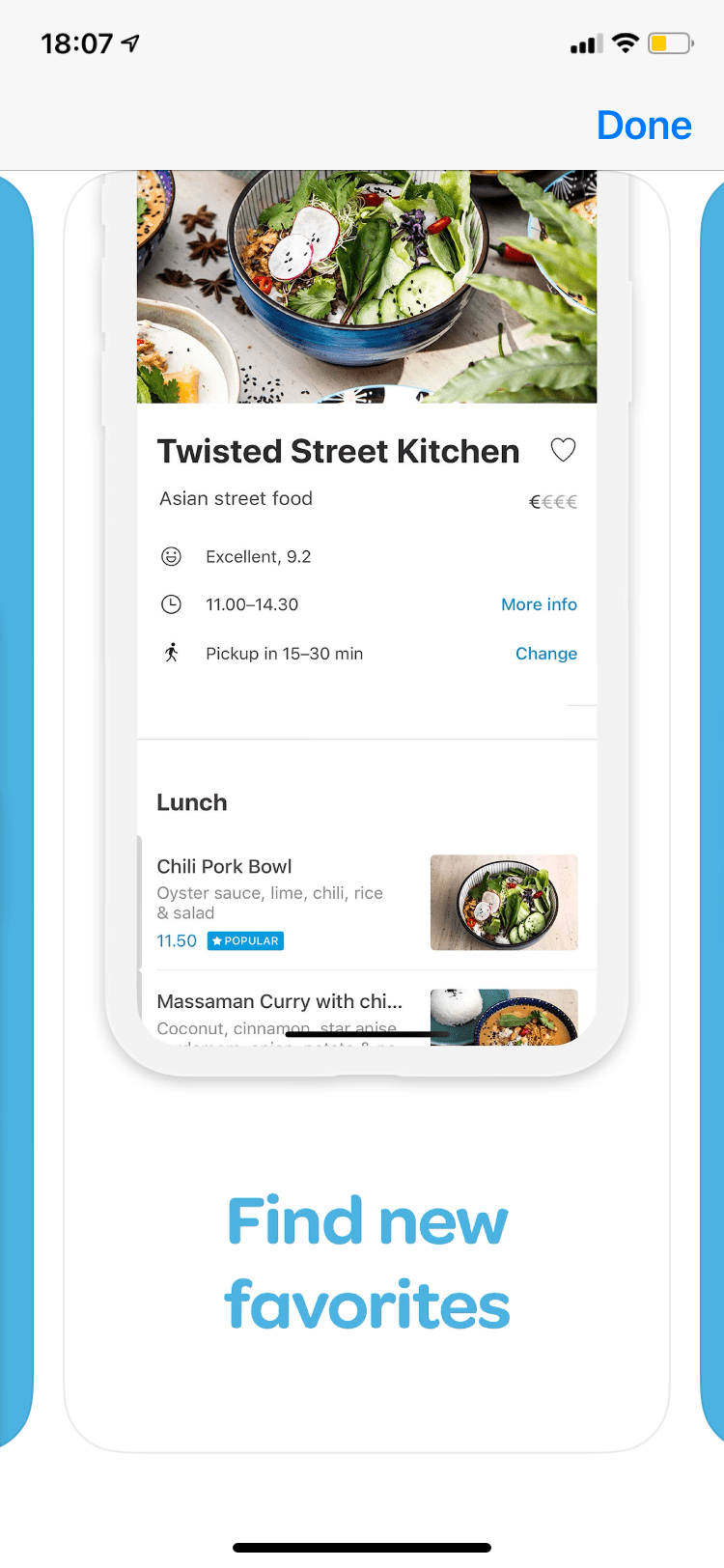The screenshot appears to be from a food website or app. At the top left corner, the time displayed is 18:07, while the top right corner shows the signal icons: data, Wi-Fi, and a battery icon that is halfway filled and colored yellow.

In the center of the screen, the name "Twisted Street Kitchen" is prominently displayed. Above the name, there is an image of a bowl containing sliced radishes, cucumbers, and some type of lettuce.

Below the restaurant name, the text "Asian street food" is displayed. The restaurant has an excellent rating of 9.2 out of 10. The operating hours are listed as 11:00 to 14:30, with a pickup time of 15 to 30 minutes.

The menu items include:
- Lunch Chili Pork Bowl: Oyster sauce, lime, chili, rice, and salad for $11.50.
- Wasa Man Curry with Chicken: Contains coconut, but the rest of the description is cut off.